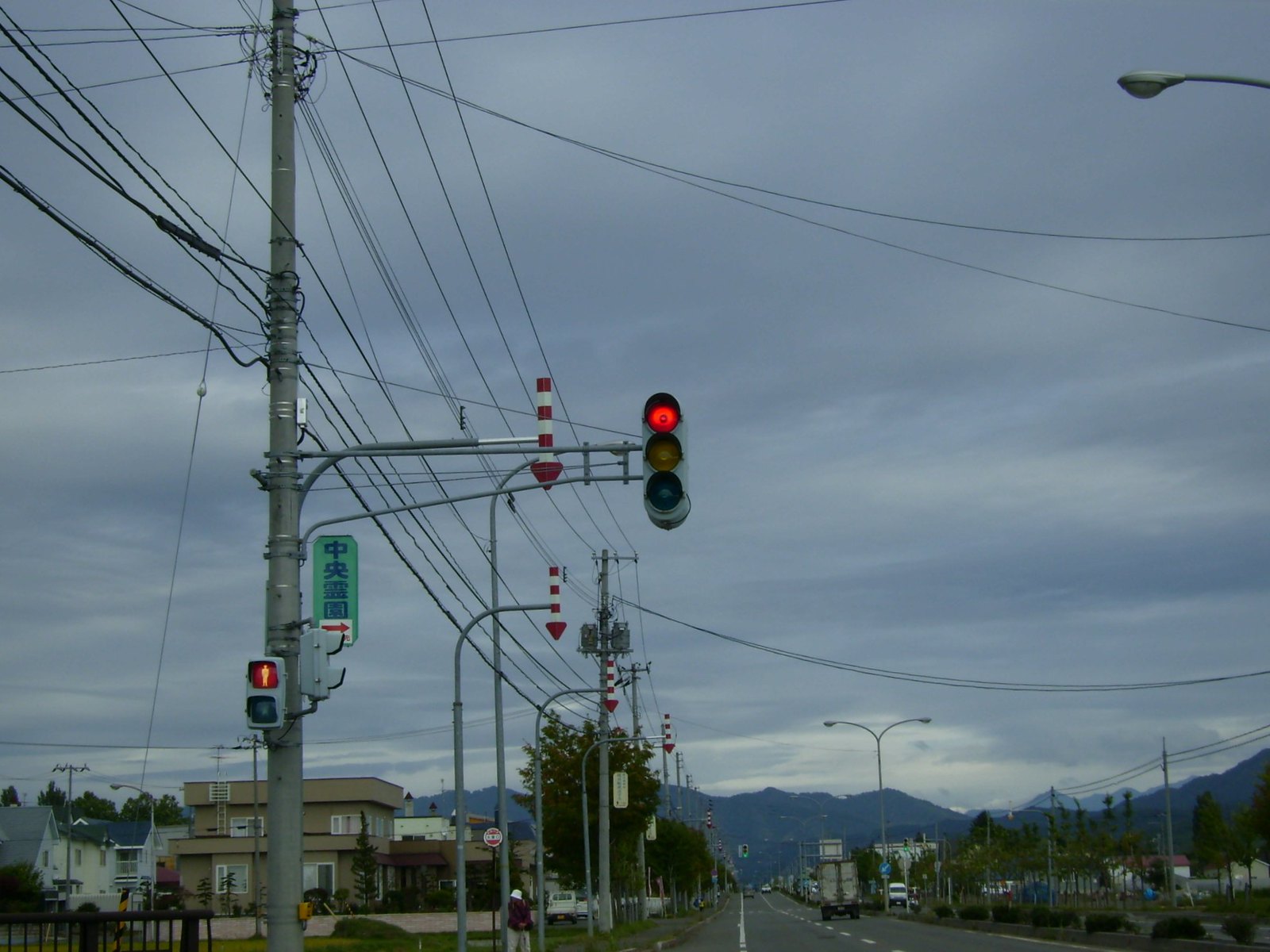The photograph captures a street scene in an Asian town surrounded by mountainous terrain. The sky is heavily overcast, casting a gloomy light over the area. Central to the image is a tall gray metal pole with numerous power lines and a traffic light that is currently red. Below the traffic light, a pedestrian walk sign also glows red. The street is a two-lane road with visible white lines, and a few vehicles, including an 18-wheeler, can be seen traveling on it. Lining the street are tan buildings and trees with leaves, and there are additional small businesses and homes visible on the right. The background showcases distant mountains, some of which appear snow-capped and shrouded in low, thick clouds. A green rectangular sign with Asian text and an arrow is also affixed to the pole. Additionally, red and white cones are attached to the wires, likely for aviation safety. The overall atmosphere suggests a gray, possibly stormy day, contributing to the scene's somber tone.